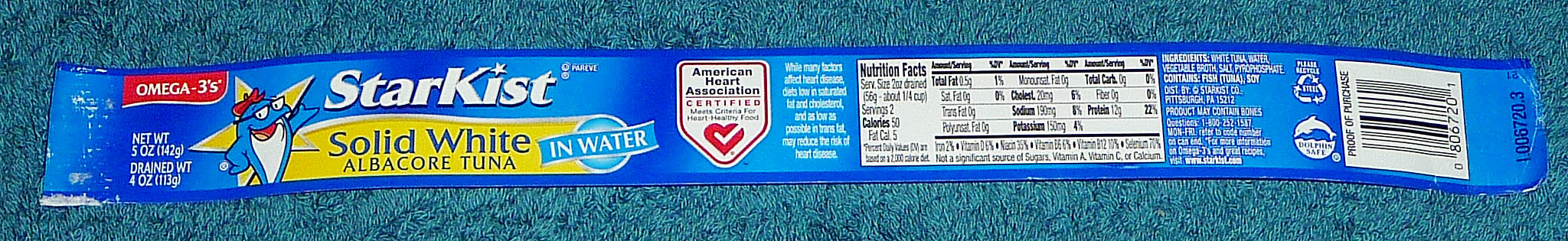This is a label for Starkist Solid White Albacore Tuna, meticulously peeled off from the can and laid out flat. Dominantly featuring a medium shade of blue, the label showcases the white 'Starkist' logo prominently. Central to the design, a yellow banner highlights the product name in bold blue text: "Solid White Albacore Tuna in Water," underscoring its premium quality. To the left, the affable Starkist mascot, a smiling tuna in glasses and a red hat, stands proudly with one hand on its hip and the other extended. Accompanying this, a red marker above the mascot declares the presence of Omega-3s, and the label is certified by the American Heart Association for heart health. To the right, essential nutritional information and a barcode complete the label layout, although they aren't clearly legible due to the image's quality. The label rests on a bluish, splotchy countertop that complements its dominant hues.